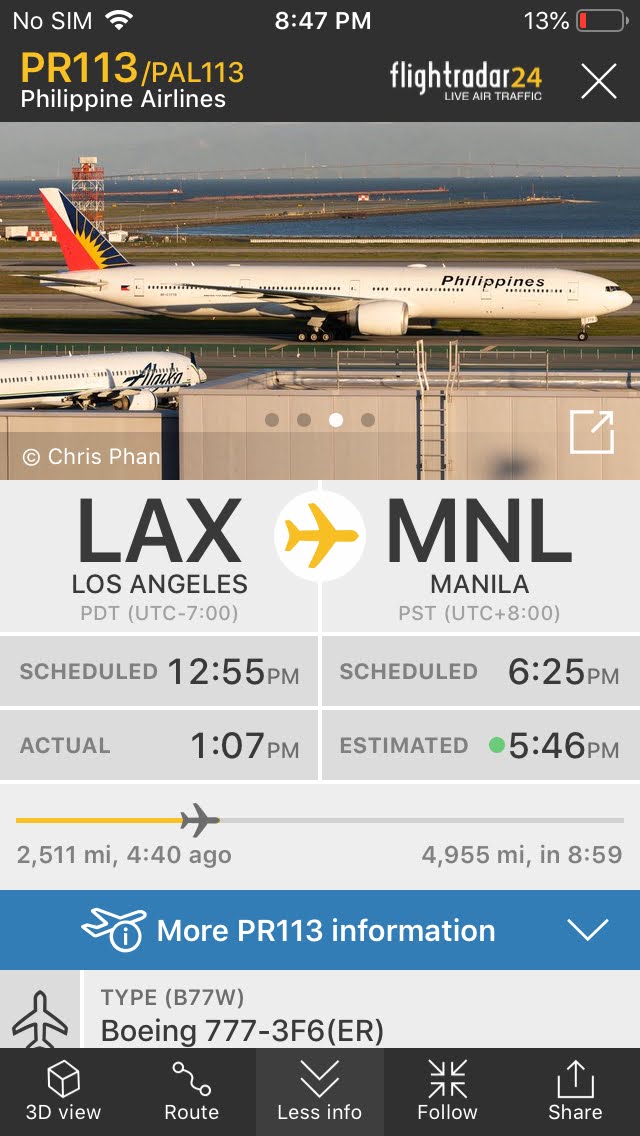At 8:47 p.m., with 13% battery remaining, a screenshot from FlightRadar24 displays Philippine Airlines (PAL) flight PR 113, a Boeing 777-3F6(ER), on the tarmac at Los Angeles International Airport (LAX). The flight is en route to Ninoy Aquino International Airport (MNL) in Manila. Originally scheduled to depart at 12:55 p.m., it was rescheduled to 1:07 p.m. and is now estimated to leave at 5:46 p.m. The total distance of the flight is 7,456 miles, with 4,955 miles left to travel and 2,511 miles already covered.